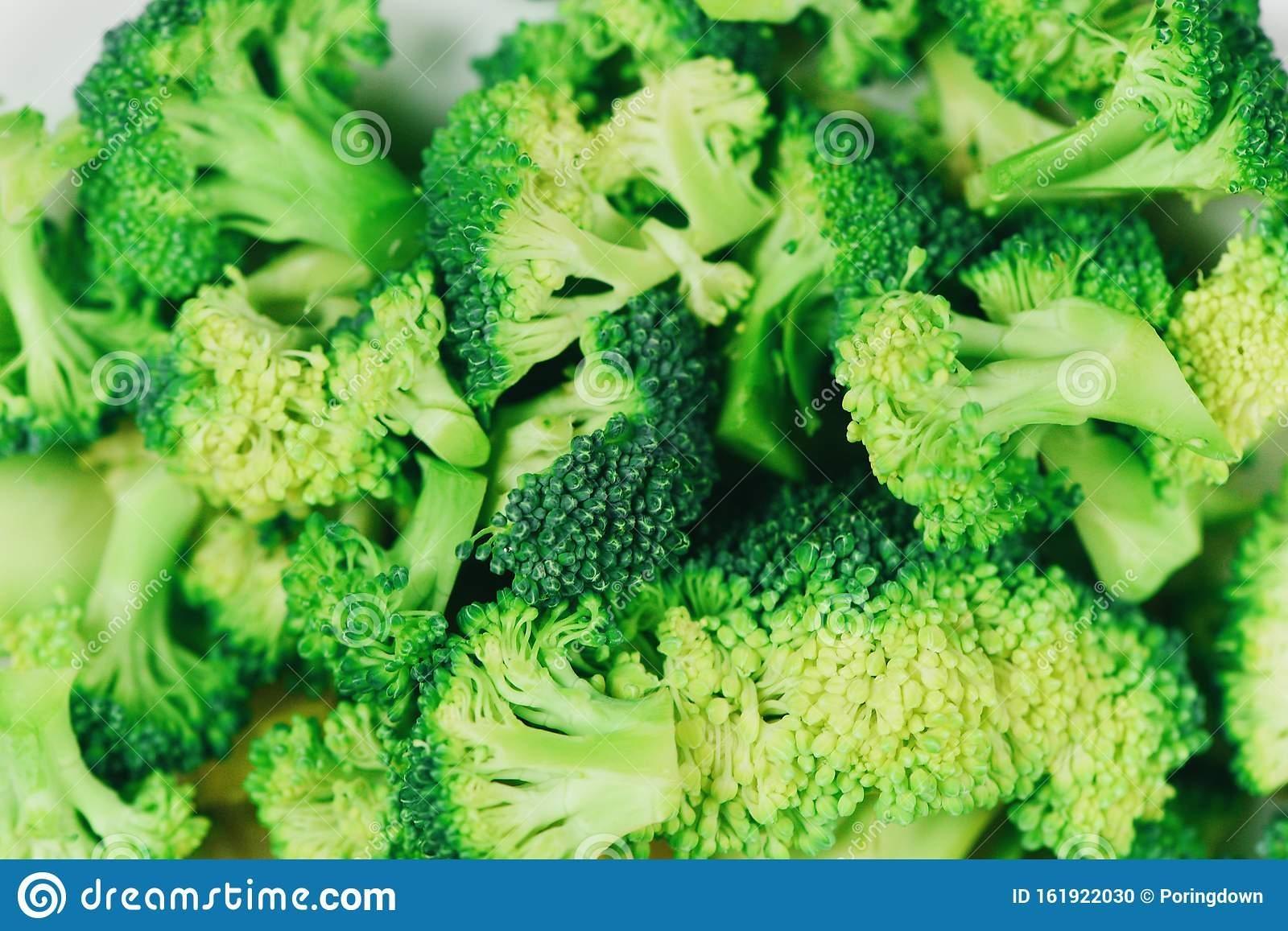This is a detailed, overhead, close-up photo of lightly cooked broccoli florets arranged on a white plate, with a striking contrast between the dark green tops and light green stems. The broccoli appears freshly blanched, showcasing a range of green shades from dark in the middle to lighter at the edges, with some florets cut in half, revealing the internal texture of the vegetable. Covering the image is a watermark made up of criss-crossing lines and a recurring swirl design, reminiscent of Naruto's insignia. It reads "Dreamstime.com" diagonally from the bottom left to the top right in four lines. At the bottom of the photo is a thin blue banner with a white spiral design in the left corner, accompanied by the white text "Dreamstime.com". In the bottom right corner, smaller white text reads "ID 161922030" followed by "Porrington Down".